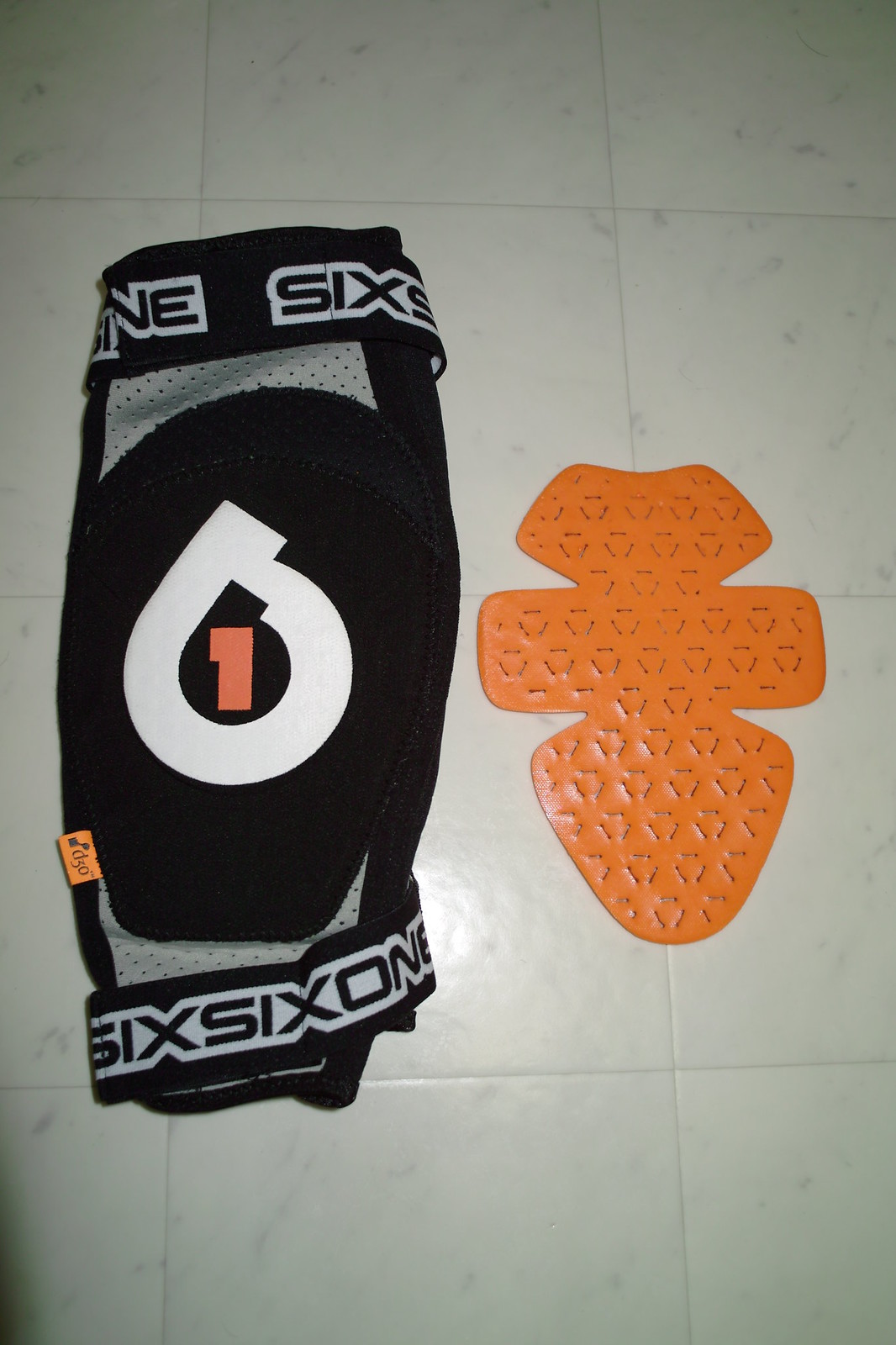This photograph features a black knee pad, likely designed for athletic use, placed on a white marble tile floor with subtle gray specks. The knee pad comprises two black straps at the top and bottom, each displaying the text "SIXSIXONE" in black letters. Prominently featured in the center of the knee pad is a bold white number "6," within which a black number "6" is nested, enclosing an orange "1" at its core. Surrounding this central design are sections of gray mesh fabric, interspersed with the black padding. There is also a small orange tag on the left side of the knee pad. To the right of the knee pad lies a segmented orange plastic insert, consisting of three shapes: a somewhat square design at the top, followed by a rectangular section, and finishing with an oval shape with rounded edges. These elements jointly illustrate the knee pad's detailed design and accompanying components.